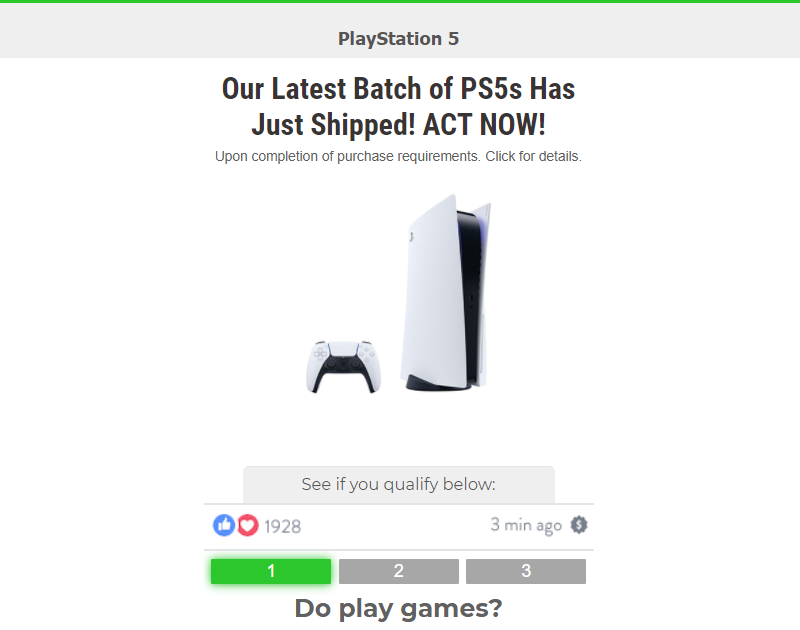Here's a detailed and descriptive caption for the image:

---

"Presenting our latest shipment of PlayStation 5 consoles! In this freshly dispatched batch, the PS5 stands out with its sleek black and white design, accentuated by subtle blue lighting that gives it an ultra-modern appearance. Currently boasting 1,928 likes, this post seems to be a hit among our followers.

In the image, there is an eye-catching element where the question 'Do you play games?' is displayed, with 'Yes' highlighted in green and 'No' and 'Not Yet' in gray. The overlay indicates this exciting update was posted just three minutes ago, showing the real-time engagement with our community.

Additionally, there’s a noticeable grid at the top of the image, traversed by dynamic green lines, adding a futuristic touch. There's also a dollar sign next to an exclamation mark, suggesting some sort of promotional offer. 

Don’t forget to check if you qualify for our latest offer and elevate your gaming experience with the new PS5 from this superbly crafted and environmentally detailed batch!"

---

This caption includes all the specifics while making it engaging and detailed for viewers.